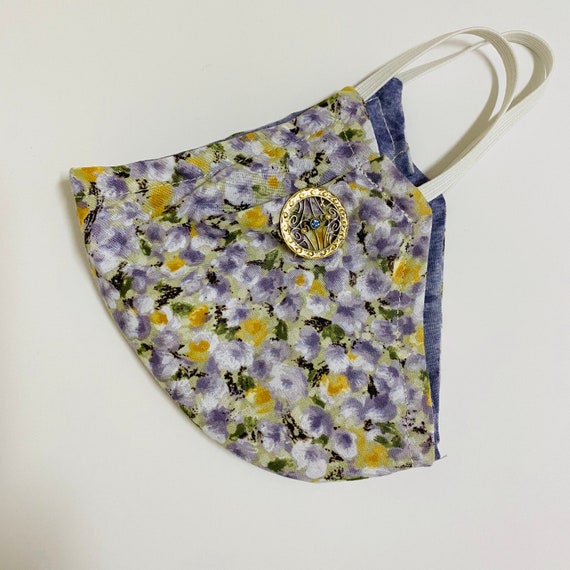The image depicts a folded, floral-patterned face mask placed diagonally on a plain white surface, likely a table. The mask's right side features a white strap extending toward the upper right, casting faint shadows. The material appears thick, possibly resembling denim or corduroy, adorned with an intricate pattern of purple and yellow flowers. Centrally positioned on the mask is a circular golden brooch with delicate scroll designs and a small blue gemstone in the middle. The overall color scheme combines violet, blue, white, gold, and yellow hues, contributing to the mask's elegant appearance.